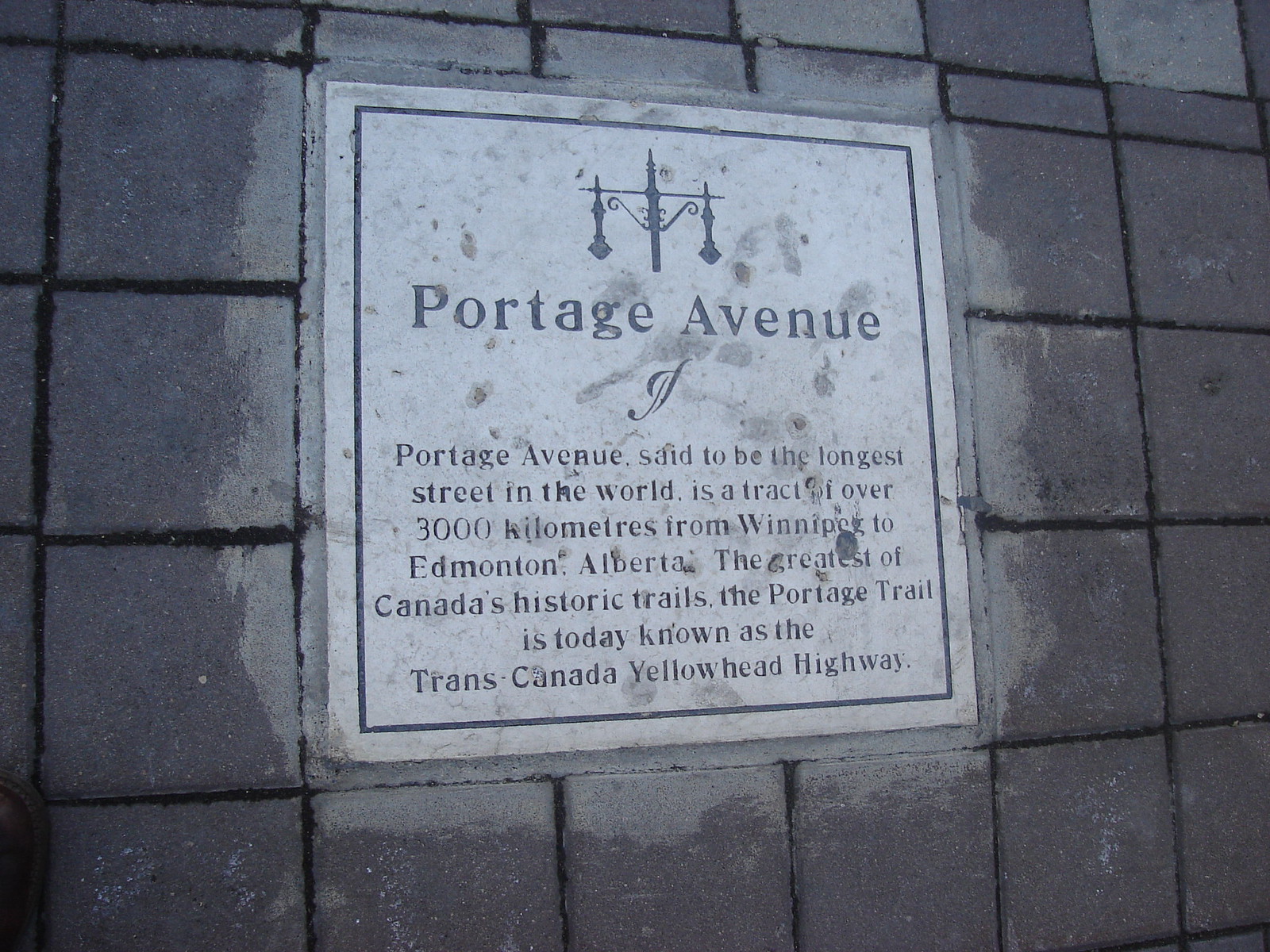This is an informative historical marker integrated into a wall of square-shaped stones, possibly the side of a building. The wall is constructed of dark, gray stone blocks. The lighter gray marker, outlined in blue, features a small design at the top resembling a decorative streetlamp or gate post. The marker reads: "Portage Avenue," and provides a detailed description below. It states that Portage Avenue is said to be the longest street in the world, stretching over 3,000 kilometers from Winnipeg to Edmonton, Alberta. It highlights Portage Avenue as the greatest of Canada's historic trails, which is now a part of the Trans-Canada Yellowhead Highway. The marker underscores the historical significance of the Portage Trail within Canada.